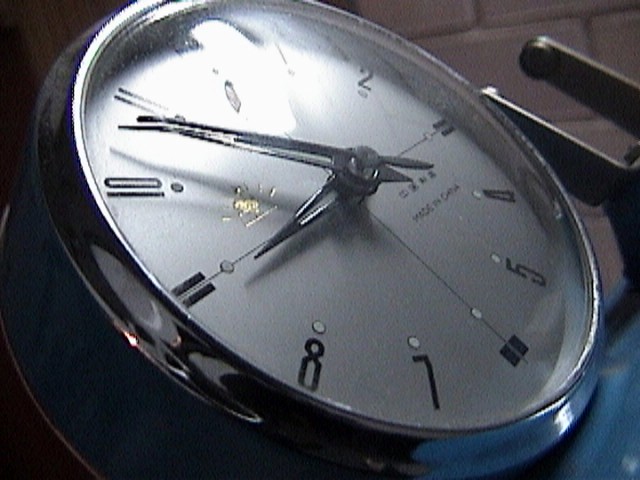The image showcases a circular wristwatch, viewed closely from the side with a detailed and slightly grainy resolution. The watch, encased in a reflective, grayish-silver or stainless steel rim, features a white or possibly pearly white face. Its clear glass cover is illuminated by a bright light, particularly near the 11 and 12 positions, obscuring some details. The clock face itself displays black numbers, though 3, 6, 9, and 12 are partially hidden due to the light reflection. The watch hands—comprising a small hour hand, a larger minute hand, and an additional second hand—indicate a time around 8:53. Under the clock hands, the text "Made in China" is prominently printed in black. The background of the image includes a dark purple tile or light purple brick wall with a gray U-shaped hook visible in the top right area, further enriching the context of the scene.